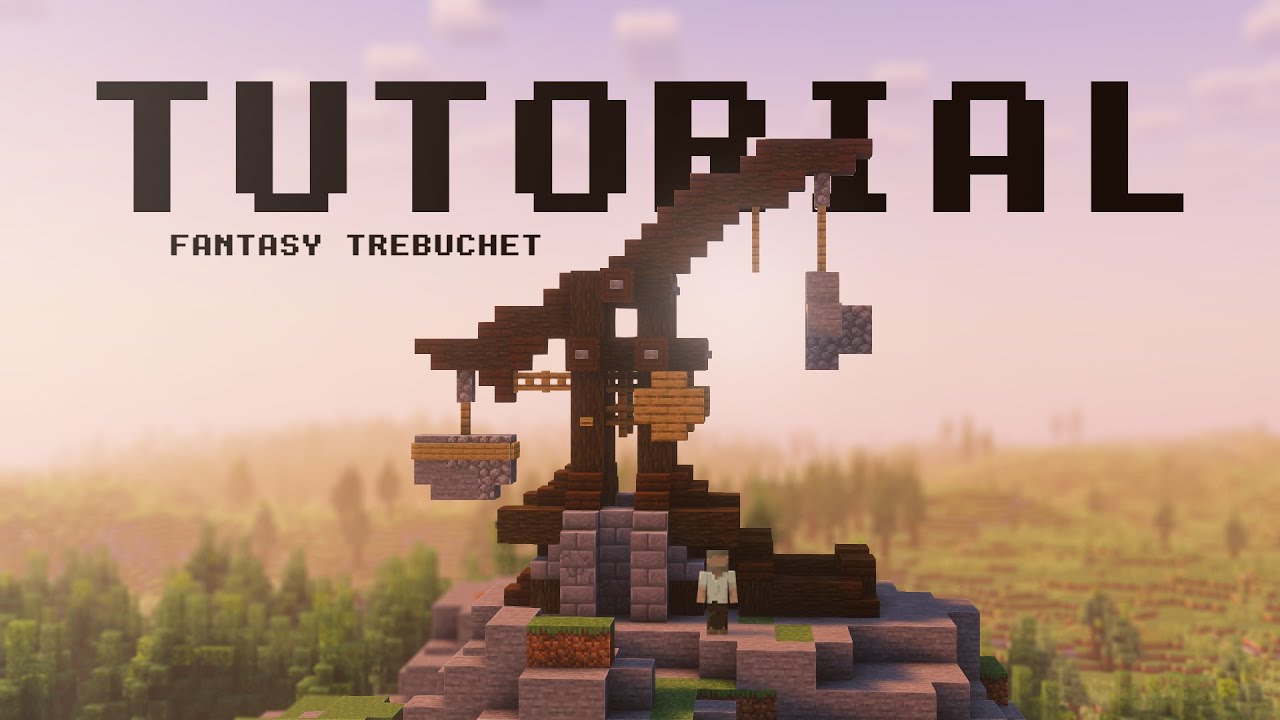The digital piece, resembling the style of Minecraft, presents a horizontally rectangular landscape that is intricately detailed yet unmistakably computer-generated. The setting is outdoors under a light purple sky, featuring a blend of digital trees and terrain blocks. The foreground showcases blocks of dirt topped with grass and stone, forming a mound. Atop this mound stands a detailed trebuchet made of wooden Minecraft blocks, with ropes and weights extending outwards. A Minecraft character with gray hair, a gray beard, a worn cotton t-shirt, and ripped brown pants stands at the base of the structure. In the background, the signature Minecraft universe with blurred trees and mountains stretches out. Bold, blocky text at the top reads "Tutorial Fantasy Trebuchet," capturing the essence of a vintage video game tutorial screen from the 1980s.